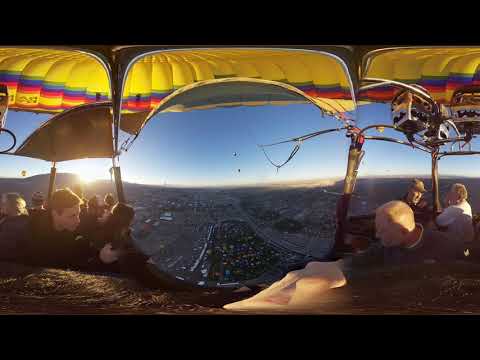This is a detailed image taken from inside a hot air balloon, showcasing a vibrant scene high above the ground. At the top of the image, you can see the colorful parachute of the balloon, predominantly yellow with stripes of blue, red, and green. The sun shines brightly from the left, casting a warm light over the spectacle. 

In the wooden basket below, multiple people, likely older, are visible. In the right section of the basket, a man with white hair sits in front, with a man and a woman behind him; the woman is dressed in white, and the man wears a ball cap. Both are partially obscured by a camera setup above them. To the left, more individuals are seated, but their features are less distinguishable. A man in the front with short hair and a dark-colored shirt can be noted.

Surrounding this scene is an impressive aerial view. Below the balloon, cars and buildings appear as tiny specks, forming a sprawling cityscape. Farther out, mountains rise majestically against a clear sky. This image radiates the essence of an adventurous, high-altitude journey in a vividly colored hot air balloon.